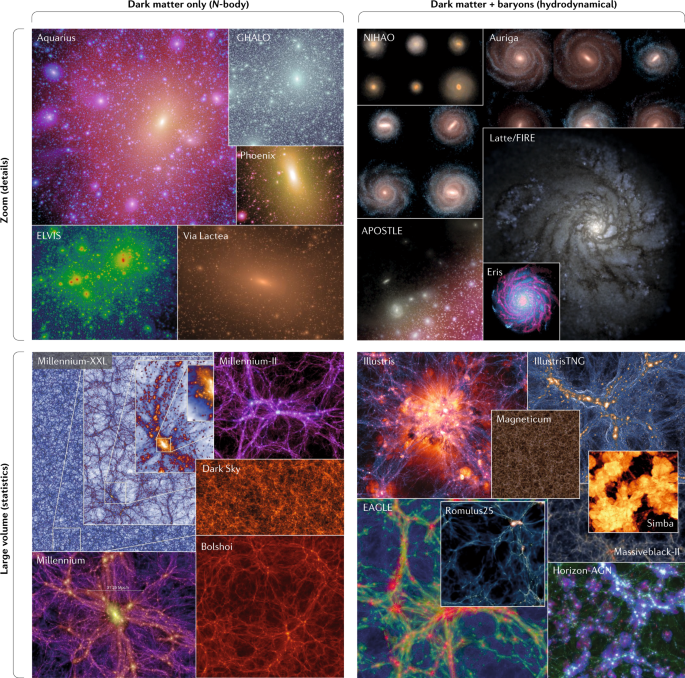This detailed image is a scientific chart divided into four quadrants, each illustrating various celestial bodies and simulations with distinct labels. The top left quadrant shows five images of celestial phenomena under the label "Dark Matter Only," including prominent objects like Aquarius, Chalo, Phoenix, Via Lactea, and Elvis. The top right quadrant is labeled "Dark Matter Plus Baryons, Hydrodynamical" and features Nehau, Aurigua, Latae, Fire, Apostle, and Eris. The bottom left quadrant, titled "Large Volumes, Statistics," presents colorful representations of vast cosmic structures such as Millennium, Dark Sky, Bal Shoi, Millennium XXL, and Bullshoy. The bottom right quadrant, possibly depicting detailed simulations or close-ups, includes notable entities like Illustrious, Magneticum, Eagle, Romulus 25, Simba, and Horizon Aegean. The chart also indicates detailed axes with terms like "Zoom Details" on the left and "Large Volume Statistics" at the bottom. Scattered across the image are vivid graphical depictions of galaxies and cosmic structures, including swirls resembling the Milky Way and clusters with a mix of yellow and blue hues.